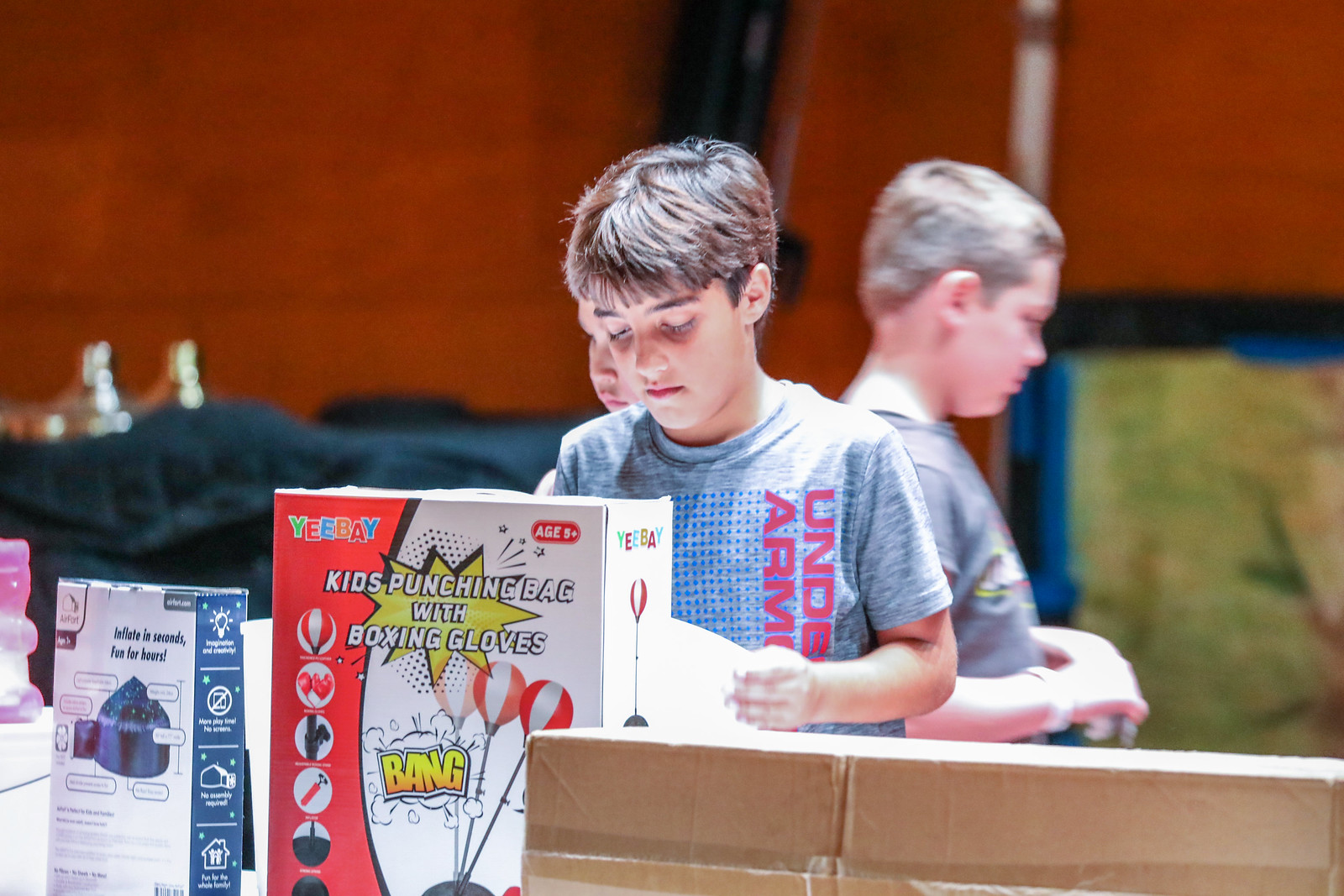The photograph depicts a group of three young boys, all appearing to be around 8 years old, gathered around a table laden with various products. The central focus is a boy with short brown hair, wearing a grey Under Armour t-shirt, intently looking at a piece of paper he is holding. To either side of him, partially visible, are two more boys. The boy to the right, with shortly cropped blonde hair, is wearing a similar grey shirt and is clasping his hands in front of him, while another boy with an obscured face can be seen further back.

In front of the boys is a table filled with cardboard boxes. Most prominently displayed is a box labeled "Kids Punching Bag with Boxing Gloves," adorned with images of the product. Another box, possibly containing a tent, stands to the left, featuring a white and blue design. The background is blurred but features patches of red, dark blue, and yellow. Despite the blur, the colorful hues provide a vibrant backdrop to the scene.